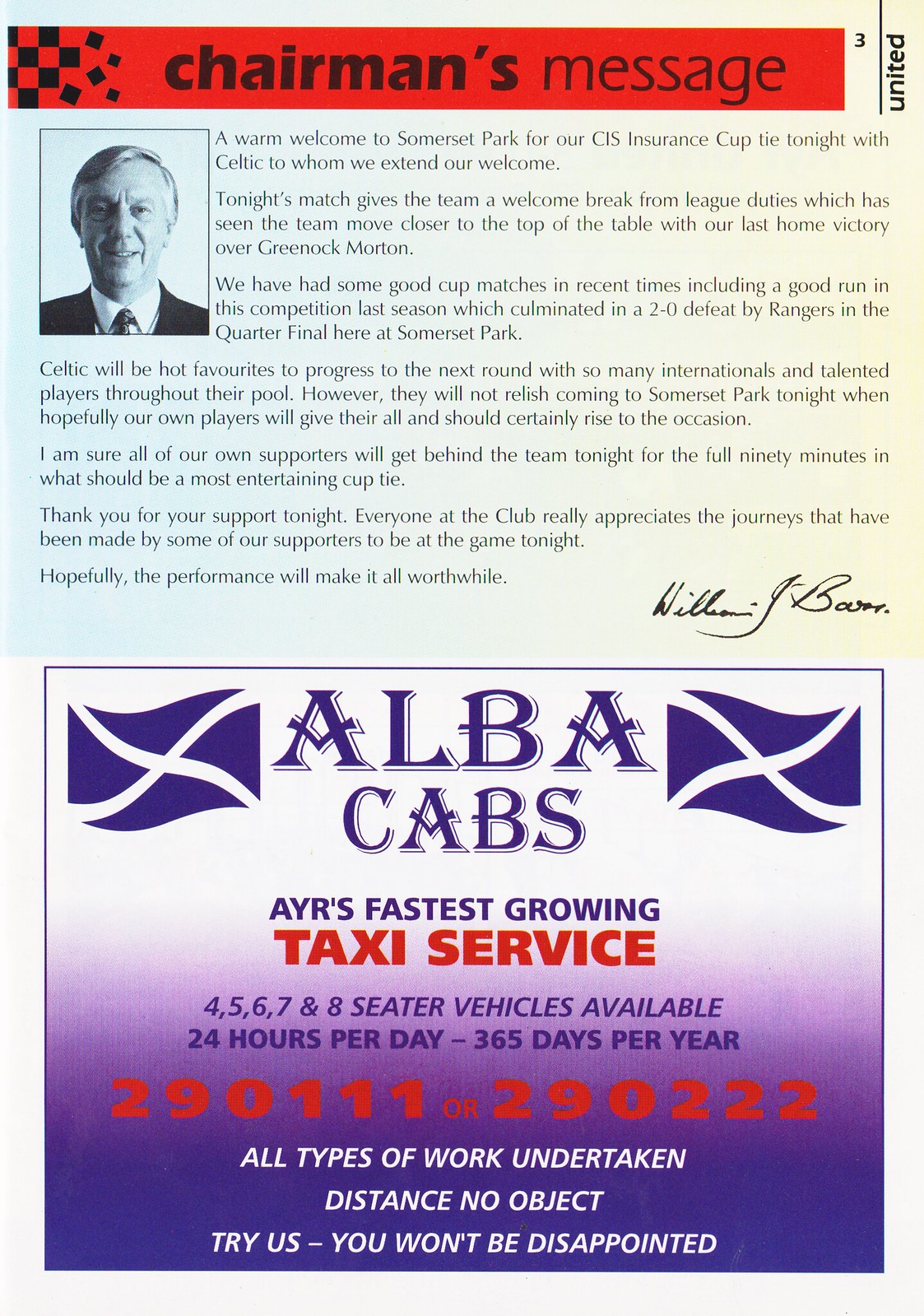This single-page pamphlet combines a warm welcome message from the chairman of an English football club with an advertisement for Alba Cabs. The top half features a vivid red banner stretching nearly across the page, with "Chairman's Message" written in bold black text. To the left, there's a black-and-white photograph of the chairman, William J. Bower, depicted from the upper chest up, dressed in a suit with a light-colored button-down shirt and tie, gazing directly at the camera. The photograph appears to overlay the chairman’s detailed message, which warmly welcomes supporters to Somerset Park for a CIS Insurance Cup tie against Celtic, expressing gratitude for the fans' efforts and highlighting the significance of the match.

Adjacent to the chairman's message, there’s a signature, likely reading William J. Bower. Transitioning to the bottom half of the pamphlet, an advertisement in a gradient design shifts from white at the top to purple at the base, promoting Alba Cabs, AYR’s fastest-growing taxi service. The ad emphasizes their availability 24/7, every day of the year, offering vehicles ranging from four to eight seats. The text boasts, "Taxi service," in prominent red letters, providing contact numbers 290111 and 290222, and assures potential customers of reliable and satisfactory service with the tagline, "Try us, you won't be disappointed." The advertisement uses a sleek, professional design with white text against a purple backdrop to communicate its offerings comprehensively.